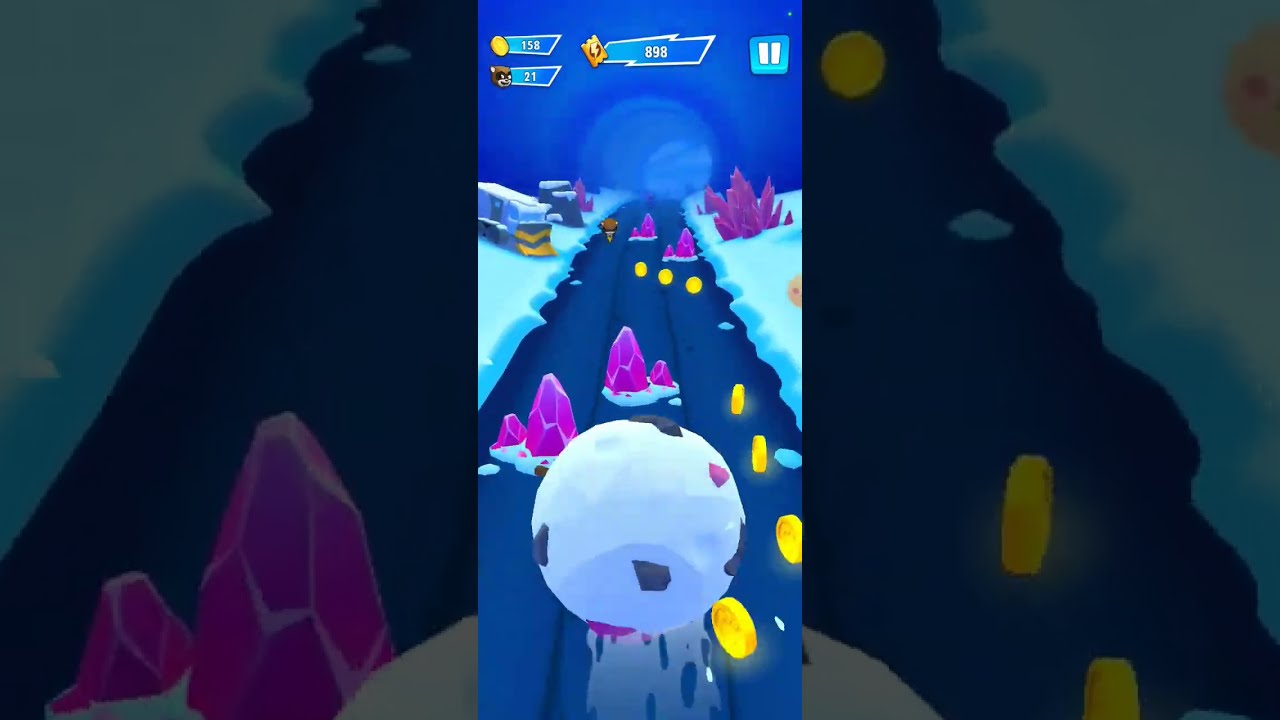This image is a detailed still from a mobile running game set in a wintry landscape. The scene features a wide, rectangular format with the middle showcasing a tall, bright screenshot of the game, while darkened close-ups of this screenshot are placed on the left and right. The central game screenshot depicts a snow-covered path with three lanes, flanked by snowbanks and featuring a river that extends towards the bottom. Rolling down this river is a large snowball adorned with purple and gray rocks, navigating around pink stones and collecting yellow coins scattered along the path. In the distance, the path continues, though the details are indistinct. Atop the image, there is a blue sky visible on the horizon, and game UI elements are displayed, including a pause button, a coin counter showing 158 coins, a ticket counter displaying 898 tickets, and a small character icon with the number 21 beside it. The goal is to avoid obstacles and gather coins, providing an immersive and dynamic gaming experience similar to the popular "Subway Surfer" style.